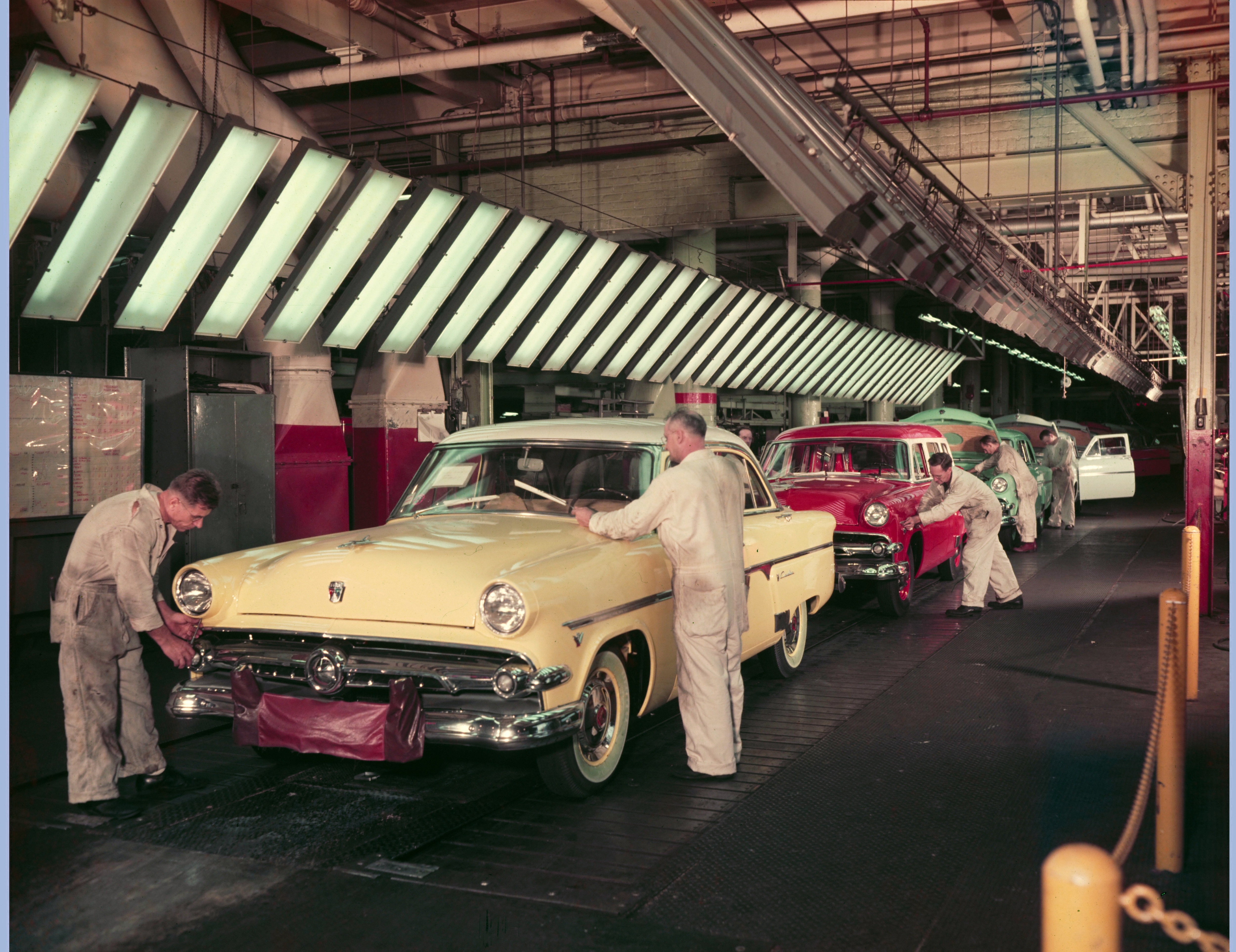The image depicts a busy auto shop scene from the late 80s or early 90s, captured on analog film. The setting is a warehouse with exposed infrastructure, including pipes, wiring, and concrete walls with red metal fixtures. The floor is black and the cars rest on metallic platforms, suggesting an easily accessible underfloor service area. 

Five mechanics, dressed in beige jumpsuits and black shoes, are meticulously working on a lineup of four vintage cars. The first car, a yellow vehicle with a white top and teal-rimmed wheels, has two men attending to it—one adjusting the windshield wipers and another working on the bumper. Directly behind it is a red car with white window trim, being serviced by a mechanic focused on the wheel area. A green car, a striking shade though partially obscured, follows next, with another worker handling its internals. Lastly, a glimpse of a white car can be seen further in the background, with its door slightly visible. 

Above the workspace, rectangular lights illuminate the scene. A yellow metal railing with a matching chain provides a boundary within the shop. The base of a nearby concrete pillar features a distinctive red bottom and cream top, seamlessly blending functionality with the shop's industrial aesthetic.